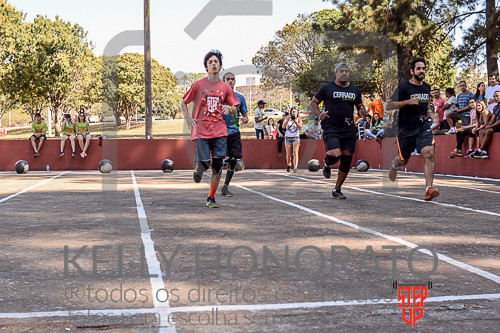The image captures a dynamic scene at a sunny track meet. Visible are at least four men in motion, each dressed in a combination of shorts, T-shirts, socks, and shoes, running towards the camera on a track delineated by multiple white lines. Notably, the runners in the two rightmost lanes wear dark shorts and dark shirts. The runner in the third lane sports blue shorts and a red T-shirt, while the competitor behind him is outfitted in darker shorts and a blue T-shirt. Each lane appears to have a ball or round object near its end. 

Surrounding the track is a small red wall beyond which a crowd is seated, their legs dangling over the edge, creating a lively spectator atmosphere. The scene is further animated by a person with a camera standing well behind the runners, capturing the event. In the background, a grassy field extends into a sparsely wooded area dotted with deciduous trees, a few pine trees, and light poles.

Across the lower section of the image, text reads "Kelly Onorato" alongside a red "Step Up" logo, suggesting ownership and possibly the purpose or theme of the event. Despite watermarks partially obscuring parts of the background, the image vividly portrays the vibrant energy and communal spirit of a track meet.